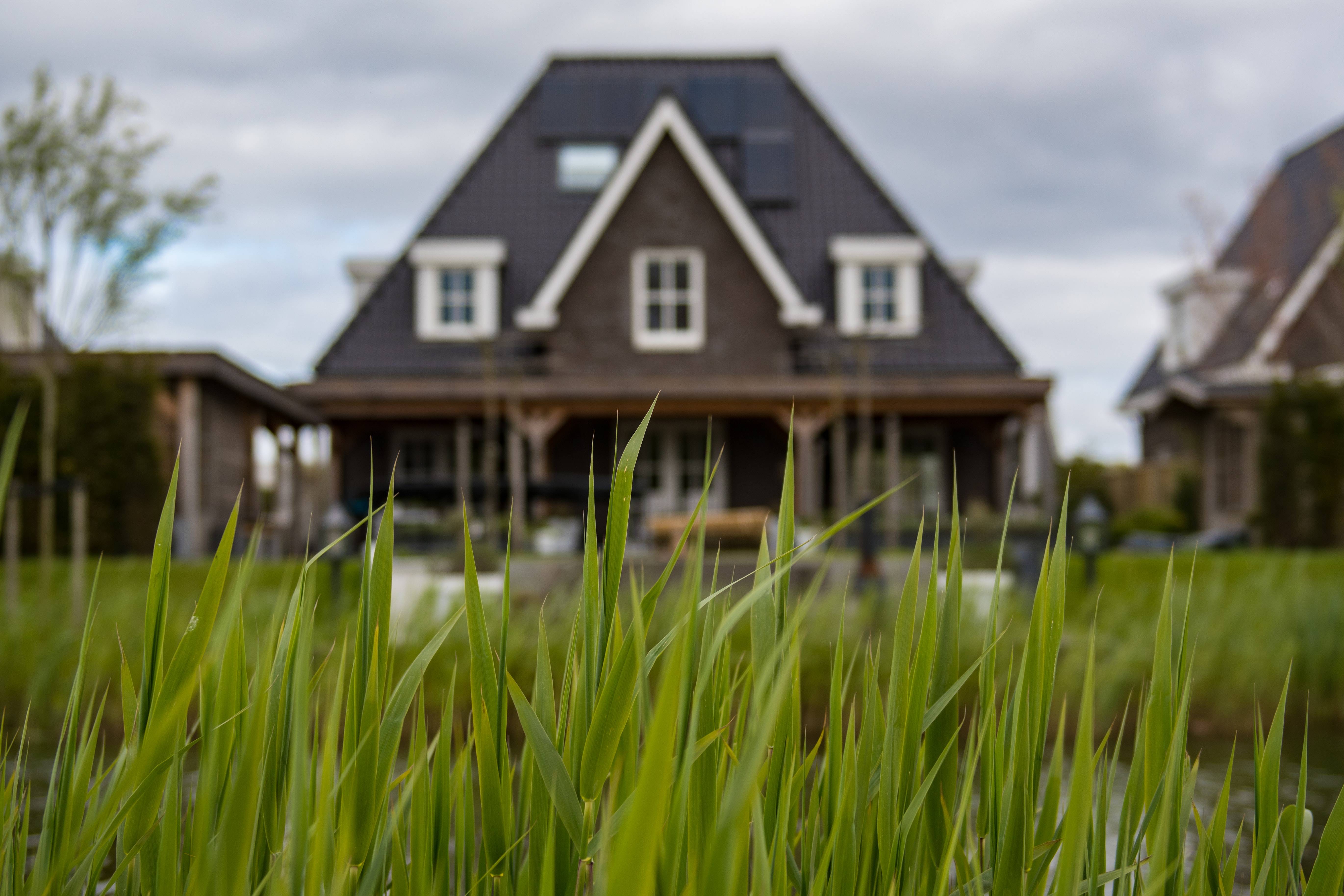This outdoor photograph captures a lush foreground of vibrant green grass blades in sharp focus, creating a striking and detailed composition. Between the blades, a small stream can be glimpsed, adding a touch of serenity to the scene. The background, slightly blurred, features a beautiful two-story house that exudes an almost idyllic charm, reminiscent of homes in the Hamptons or near a beach in the United States. This brown house with white trim and a triangular roof has a quaint porch with columns and visible white doors on the lower level. Flanking the central house are other structures, including a low, flat-roofed building on the left and another house to the right, although their details are less distinct. The sky overhead is overcast with heavy, gray clouds, adding a moody atmosphere to the otherwise picturesque setting. To the upper left, a bit of a tree is visible, further framing this tranquil yet sophisticated suburban scene.